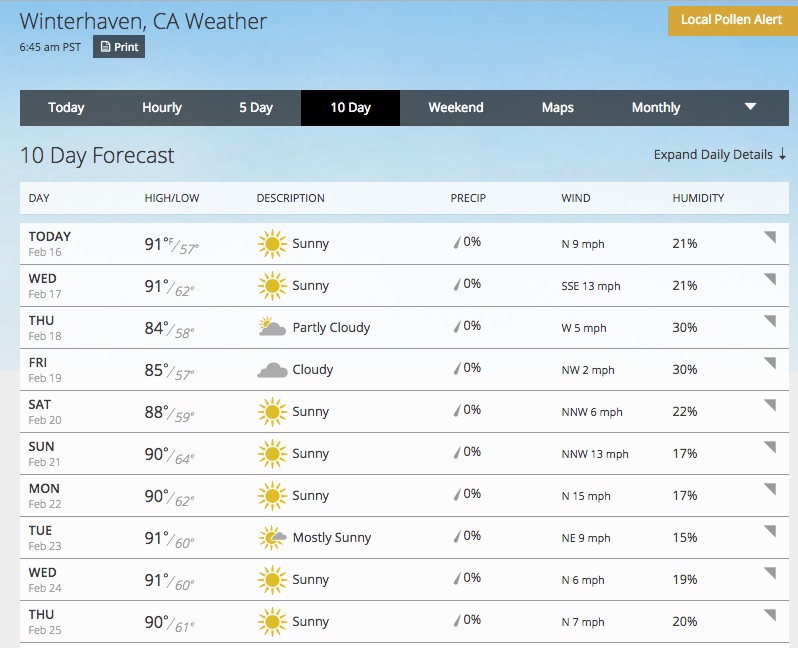Here's the detailed caption for the image description:

---

This image features a weather page from a website, predominantly utilizing a blue and white color scheme. At the top of the page, the heading indicates "Winterhaven, CA Weather," dated at 6:45 a.m. PST. Adjacent to this heading is a black rectangular button labeled "Print" in white text, accompanied by a small print icon. On the top right corner, a yellow rectangular box labeled "Local Pollen Alert" is prominently displayed.

Beneath the heading and alert, there are several navigational options for different types of forecasts and information: "Today," "Hourly," "Five-Day," "Ten-Day," "Weekend," "Maps," and "Monthly." The "Ten-Day" option is selected, highlighted in a darker shade compared to the other options.

Directly below these navigation tabs, the ten-day weather forecast is presented in a comprehensive, long rectangular box. This forecast table is organized into multiple columns: "Day," "High / Low," "Description," "Precip" (abbreviated for precipitation), "Wind," and "Humidity." The leftmost column lists the days of the week, starting from "Today" and continuing with "Wed," "Thu," "Fri," "Sat," "Sun," "Mon," "Tue," "Wed," and "Thu." For each day, weather icons depict conditions such as sunny, partly cloudy, cloudy, and mostly sunny.

---